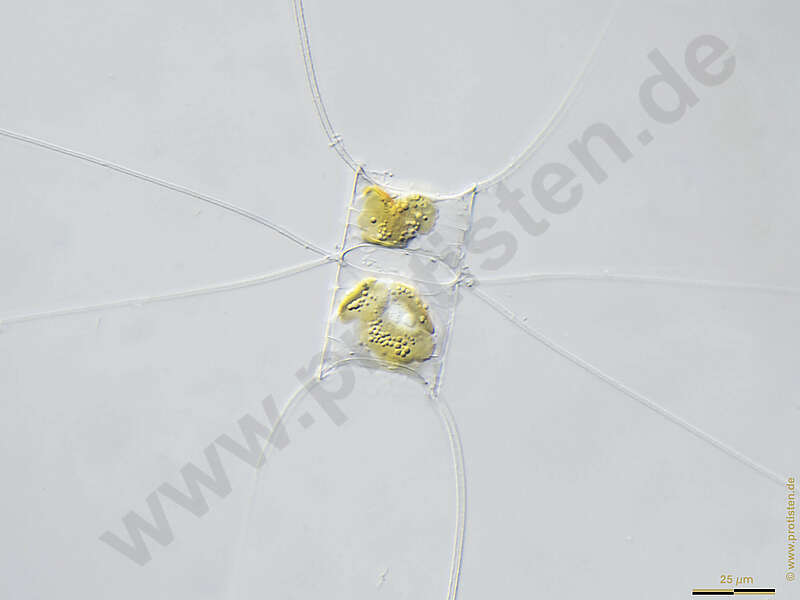The image features a textured, plaster-like background with intersecting cracks or lines that run diagonally and form an X-shape. The central focus is a rectangular area divided into two sections, each containing a gold-colored, bubbly liquid that resembles spit blobs. Overlaid diagonally across the image is a translucent but readable text that partially obscures the website URL "www.prostenten.de" or "www.protocin.de." In the bottom right corner, there is a scale marked "25mm" or "25HM" in small red text. The entire image has a blueish-gray tint, and it appears to be a prototype slide with a watermark.